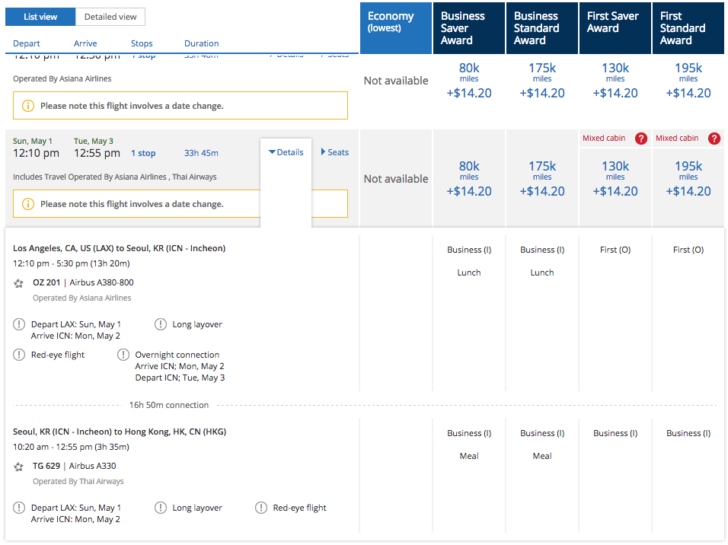The image depicts a detailed flight booking interface. In the upper-left corner, there is a blue button labeled "List View" and a white button labeled "Detail View," with the current display likely in List View mode. To the right, there's a section labeled "Choices" with options such as "Depart," "Arrive," "Stops," and "Duration." Below, the fare classes available are listed: Economy, Business Saver Award, Business Standard Awards, First Saver Award, and First Standard Award. 

Indicating that this is indeed a flight booking tool, the details mention the flights are operated by Asiana Airlines. The user can search for flights and see the required miles for various fare classes, though Economy class is not available for the highlighted options.

The specific flights available are detailed: one departing on Sunday, May 1st, arriving on Tuesday, May 3rd, crossing the International Dateline. Another segment shows a flight from Los Angeles to Seoul, departing at 12:10 PM and arriving at 5:30 PM after 13 hours and 20 minutes on an Airbus aircraft. Additionally, there's a connecting flight from Seoul, Korea to Hong Kong, departing at 10:20 AM and arriving at 12:55 PM, lasting 3 hours and 35 minutes. This implies the traveler is considering an itinerary involving a layover in Seoul before continuing to Hong Kong.